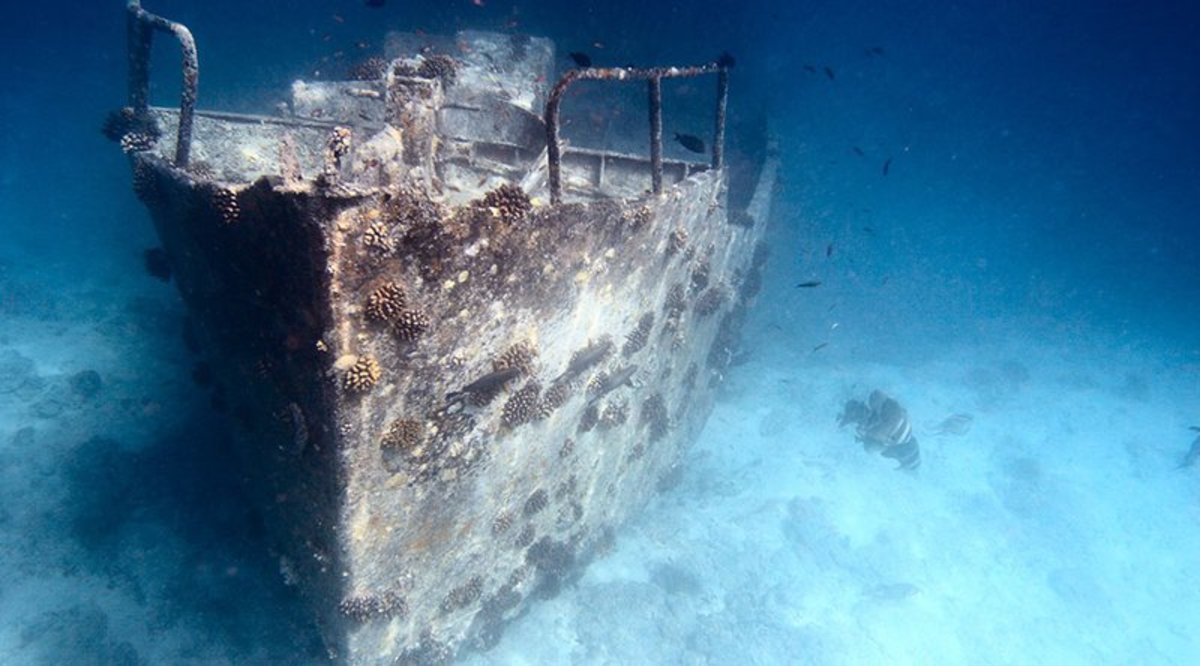This underwater photograph showcases the haunting remains of a small, sunken fishing vessel resting on the ocean floor. The scene is awash in gradients of dark, medium, and light blue, creating an ethereal underwater ambiance. The bottom is sandy with clusters of what appear to be coral or sponges growing sporadically. The vessel's weathered and rusty shell is encrusted with numerous barnacles and crustaceans, evidence of its long submersion. Guardrails on either side are visible, heavily adorned with marine life. The ship's gray and whitish hues blend seamlessly into the surrounding marine environment. Swimming among the wreckage are several fish, some with distinctive stripes. The vessel itself seems to blur into the distance, its middle and back portions fading into the deep blue water, leaving only its well-worn front clearly visible.